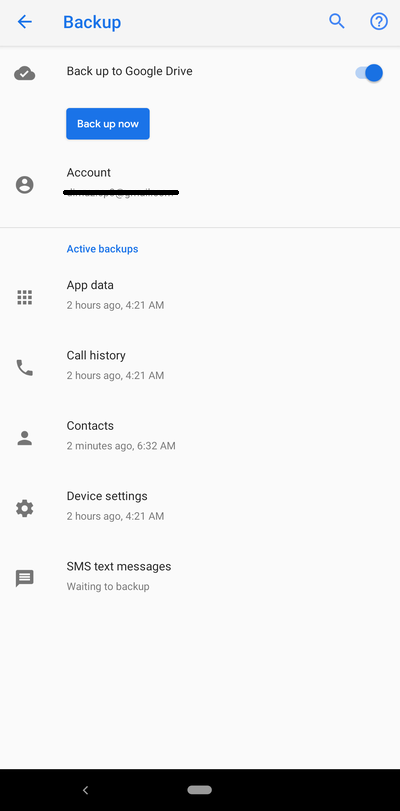The image depicts a phone interface with the title "Backup" in blue at the top, accompanied by a blue arrow pointing to the left. On the top right corner, there is a magnifying glass icon and a question mark enclosed in a circle. The main section of the screen displays the heading "Backup to Google Drive," showing a gray cloud icon with a check mark inside it.

Below this, there are two blue buttons: a smaller one on the right side and a larger rectangular button that reads "Backup now" in white text. Further down, the section titled "Account" is shown, where the account name is obscured by a black stripe. To the left of this, there is a generic gray profile icon.

The next section is titled "Active backups" in blue text. Listed under this section are various items with their respective icons to the left:

- **App Data:** Represented by a dotted icon, backed up two hours ago at 4:21 a.m.
- **Call History:** Represented by a phone icon, backed up two hours ago at 4:21 a.m.
- **Contacts:** Represented by a person icon, backed up two minutes ago at 6:32 a.m.
- **Device Settings:** Represented by a gear icon, backed up two hours ago at 4:21 a.m.
- **SMS Text Messages:** Represented by a speech bubble icon, currently waiting to be backed up.

Each item is accompanied by the timestamp of the last successful backup, providing a detailed overview of the backup status for the different data categories.